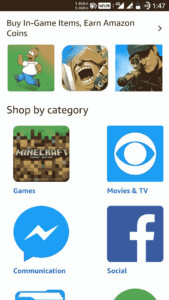**Caption:**

A screenshot of a promotional banner from the Amazon App Store, showcasing an offer to "Buy in-game items, Earn Amazon Coins." The visual includes several iconic figures such as Homer Simpson with his mouth open and a character aiming down a rifle. Below the promotion, there's a section titled "Shop by Category" displaying various categories like Minecraft, Movies & TV, Communication, and Social, each represented by distinct logos and icons of apps. The background is predominantly white with brown text, and the top part of the interface imitates an Android UI bar, also in brown.